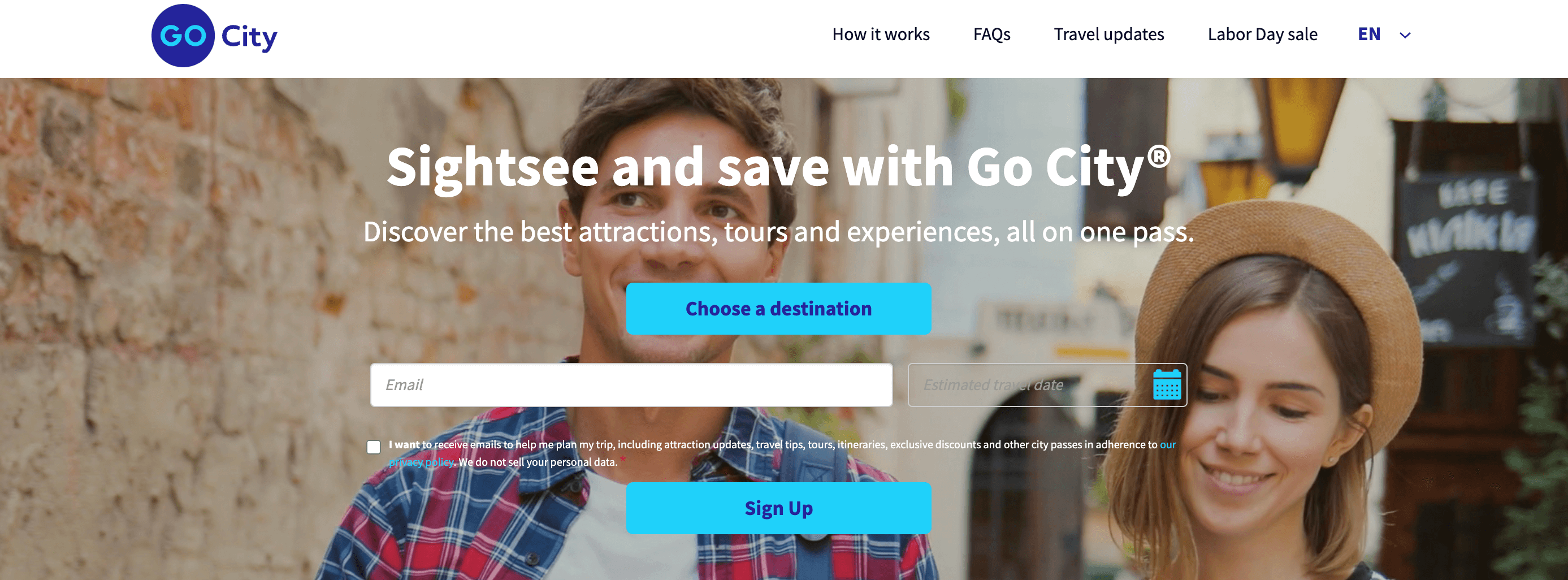This is an image from the GoCity website. In the top left corner, there is the GoCity logo, with the word "Go" inside a blue circle, colored in teal, and "city" in navy print. Across the top of the page, there are clickable sections that read: "How it works," "FAQs," "Travel Updates," "Labor Day Sale," and a language option marked "ENG" for English. 

Below the navigation bar, prominently displayed in the main section of the website, there is a photograph of a man and a woman standing in front of an old, slightly dilapidated brick wall with streetlights visible in the background. The woman, who has brown hair and is smiling while glancing down, is wearing a hat. The man, who also has brown hair and is wearing a hat, dons a plaid blue and red shirt over a t-shirt and is looking forward with a smile. Overlaying the image in white print is the text: "Sightsee and save with GoCity." Below this text, there are options to choose a destination and to sign up, both highlighted in teal.